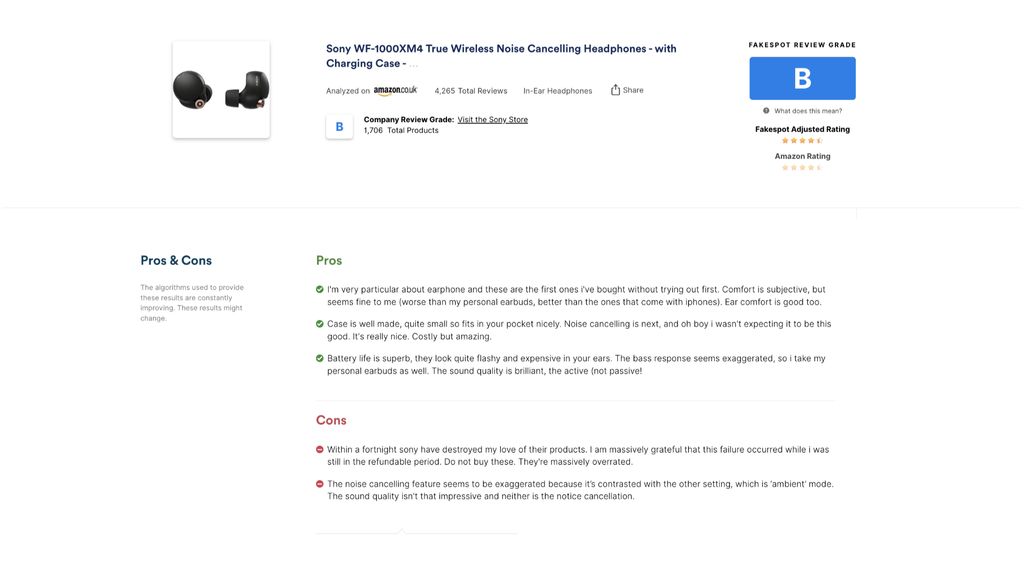**Product Review: Sony WF-1000XM4 True Wireless Noise Cancelling Headphones**

*Image Description: Featuring a pair of sleek, black earbud-style headphones, positioned in the upper left-hand corner along with their compact charging case.*

**Product Overview:**
- **Product Name:** Sony WF-1000XM4 True Wireless Noise Cancelling Headphones
- **Charging Case Included**
- **Platform:** Analyzed on Amazon.co.uk
- **Reviews:** 4,265 customer reviews in earphones category
- **Grade:** Variable
- **Store:** Visit the Sony store, featuring 1,706 total products

**Pros:**
- **Initial Impressions:** As someone very particular about earphones, these were the first pair I purchased without prior testing.
- **Comfort:** Subjective but generally acceptable. More comfortable than iPhone earbuds, though not as much as my personal favorites. Ear comfort is also commendable.
- **Case Design:** Well-made and compact, fitting nicely into pockets.
- **Noise Cancelling:** Exceptional performance, exceeding expectations. Worthwhile investment despite high cost.
- **Battery Life:** Superb longevity.
- **Aesthetics:** High-end, flashy appearance when worn. However, appears expensive.
- **Sound Quality:** Brilliant, engaging sound. The bass response is noted to be somewhat exaggerated for personal preference.

**Cons:**
- **Durability:** Product failed within a fortnight, leading to significant disappointment. The failure occurred within the refundable period, causing regret.
- **Value:** Deemed massively overrated by the reviewer.
- **Noise Cancelling:** Perceived as exaggerated due to the ambient mode contrast; not as impressive as expected.
- **Sound Quality:** Ultimately, the sound quality did not meet the heightened expectations.

In conclusion, while the Sony WF-1000XM4 headphones boast outstanding noise canceling capabilities and battery life, along with a stylish design, they also come with significant drawbacks related to durability and actual audio performance, leading to a mixed overall impression.